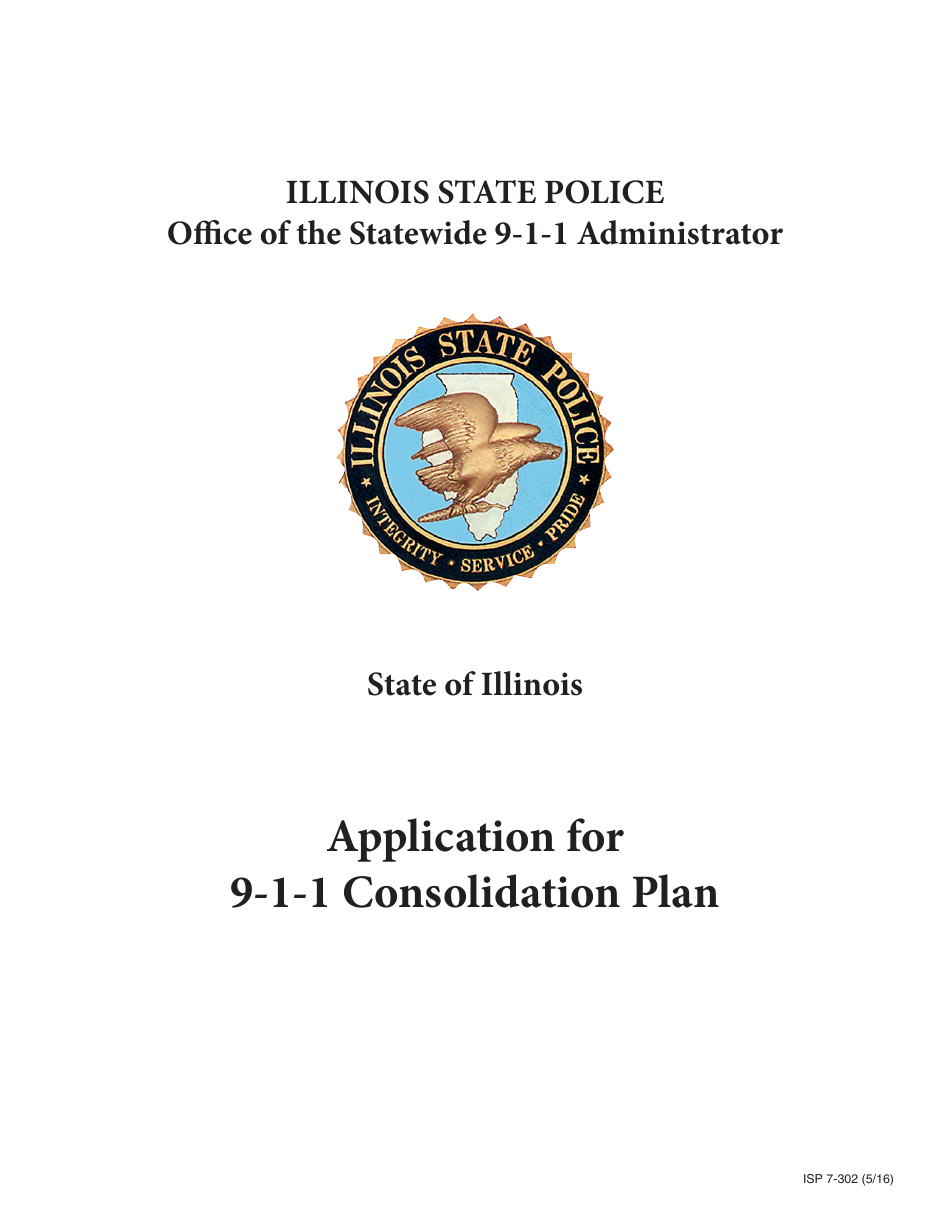The image depicts a document or a digitized form against a solid white background with no borders. At the top, it reads "Illinois State Police" followed by "Office of Statewide 911 Administrator." Below this text, centered on the page, there's a circular emblem representing the Illinois State Police. The inner circle of the emblem is blue, featuring the state outline of Illinois and an eagle facing left. The black outer part of the emblem bears the words "Integrity, Service, and Pride."

Below the emblem, the text "State of Illinois" is centered. Further down, in a slightly larger font, the document title reads "Application for 911 Consolidation Plan." In the bottom right corner, there’s small text that says "ISP 7-302-5-16."